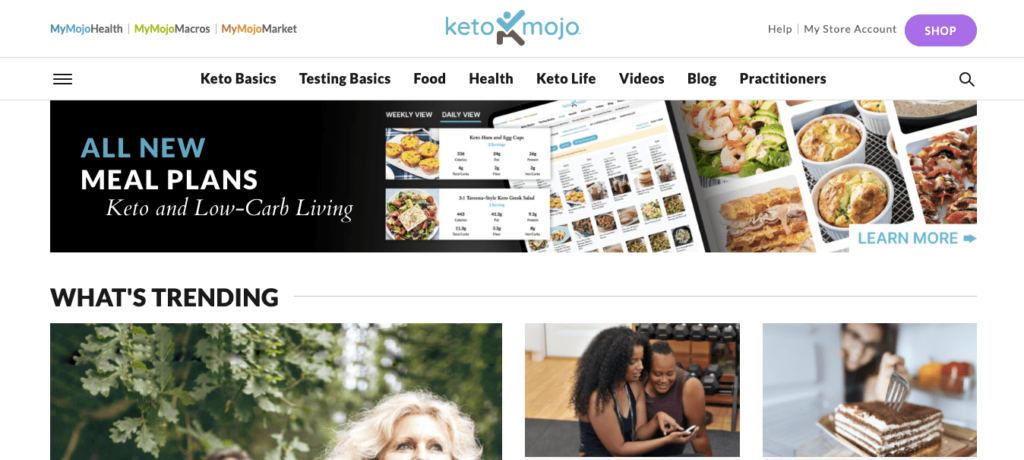This image depicts the website of Keto Mojo, a platform dedicated to supporting individuals on a ketogenic and low-carb lifestyle. On the left side of the page, there’s an illustration of a stick figure exercising. The right section features navigation tabs labeled "My Mojo Health," "My Mojo Macros," and "My Mojo Market." Below these tabs, highlighted in purple, are options for "Help," "My Store," "Account," and "Shop."

Further down, the site offers links to essential resources titled "Keto Basics," "Testing Basics," "Food," "Health," "Keto Life," "Videos," "Blog," and "Practitioners." A prominent black box announces “All New,” with “Meal Plans” highlighted in blue and further described as suited for "Keto and Low-Carb Living." Images of food are displayed alongside these menus, encouraging users to explore more by clicking a blue "Learn More" button, complete with a right-pointing arrow.

The "What's Trending" section showcases three images: one of a blonde woman surrounded by lush greenery, another of a Black man and woman examining an iPhone together, and the last one featuring a stack of square pancakes. The pancakes are topped with an unknown substance, and a hand is seen reaching out, fork poised to take a bite.